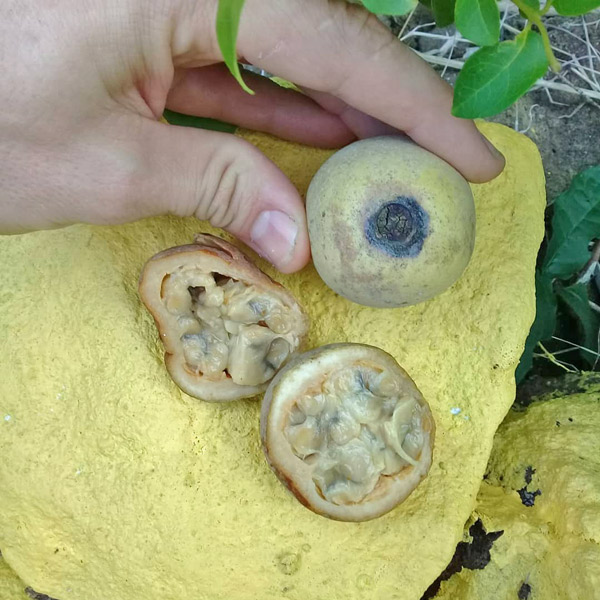The photograph showcases a close-up of a Caucasian left hand holding an oval-shaped fruit, about the size of a mandarin orange, in the top left quadrant. The fruit has a pale greenish-yellow hue with a distinctive black spot on its tip. Just below this fruit, another identical fruit is sliced in half, revealing a creamy, yellowish, almost custard-like interior that features some irregular clumps and a somewhat gooey texture. Both fruits are resting on a large, yellow object which resembles a tortilla in texture but may also be interpreted as a rock. The background includes visible soil with trailing vines and green leaves, adding a natural setting to the photograph. Another yellow object is partially visible in the bottom right corner, enhancing the color palette and natural context of the scene.